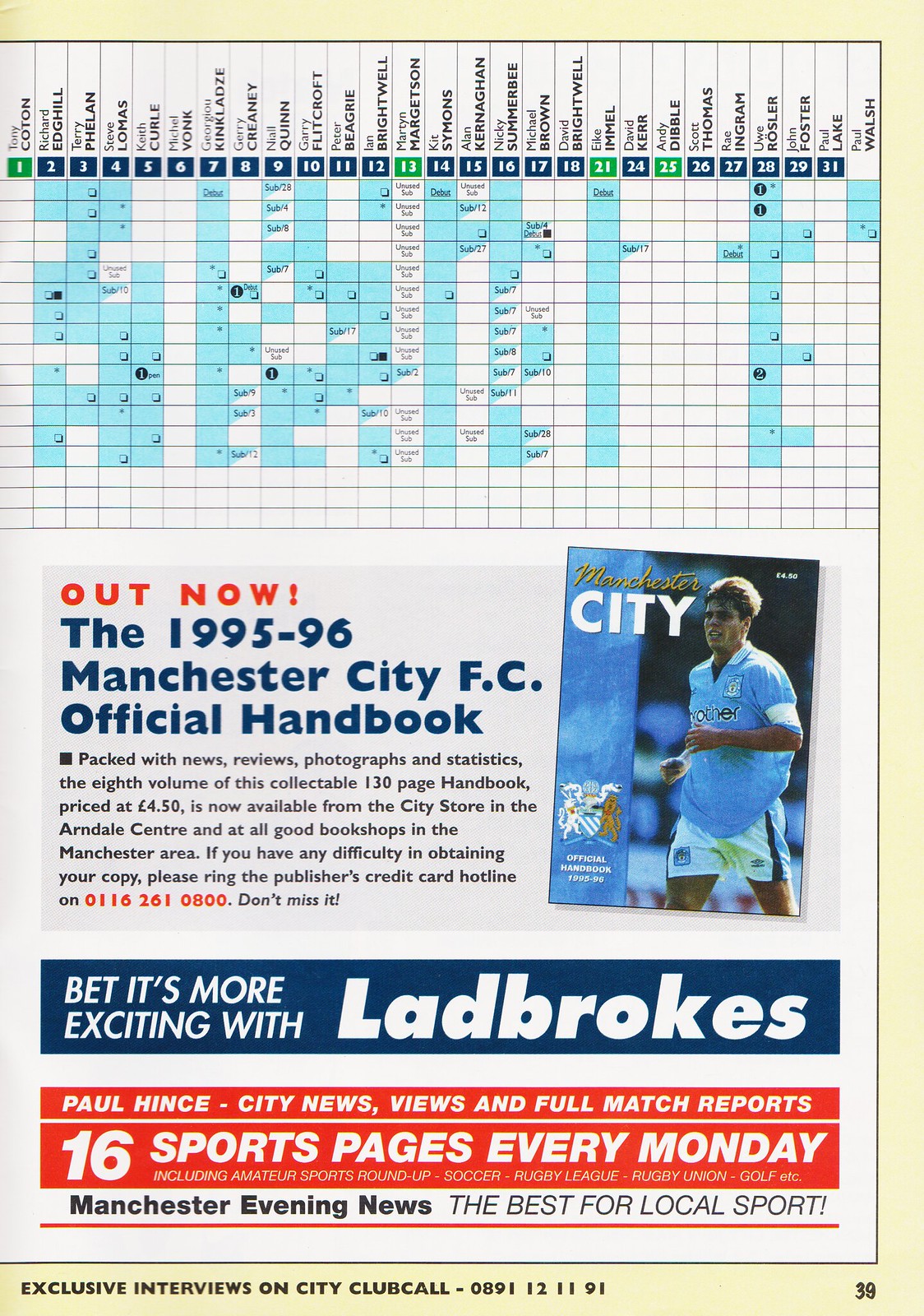The image is a scan from a soccer-related magazine or newspaper, centered on an advertisement for the 1995-1996 Manchester City FC Official Handbook. At the top, there's a sequence of numbers from 1 to 31, each paired with different names, possibly indicating player statistics or schedules. Below this, text reads, "Out now: the 1995-96 Manchester City FC Official Handbook," highlighting it's packed with news, reviews, photographs, and statistics. It is the 8th volume and consists of 130 pages, priced at £4.50, available from the City Store in the Arndale Centre and local bookshops. A contact number for the publisher's credit card hotline is 0116 261 0800 for those having trouble obtaining a copy.

To the right, there's an image of the handbook's cover, depicting a man in 90s sports attire with "Manchester City" written on it. The layout is sporty, with colors such as pale blue, white, dark blue, rich red, and yellow creating a vibrant look. 

Below the handbook's announcement, there is a banner stating, "Bet it's more exciting with Ladbrokes." Further down, a red banner reads, "Paul Hintz: City News, Reviews and Full Match Reports, 16 sports pages every Monday." The footer concludes with, "Manchester Evening News, the best for local sport," followed by a yellow-bordered callout for "Exclusive Interviews on City, Club Call 0891 121191." The number 39 is visible in the bottom right-hand corner. The overall style centers all elements and conveys a lively and engaged tone, characteristic of 90s sports designs.